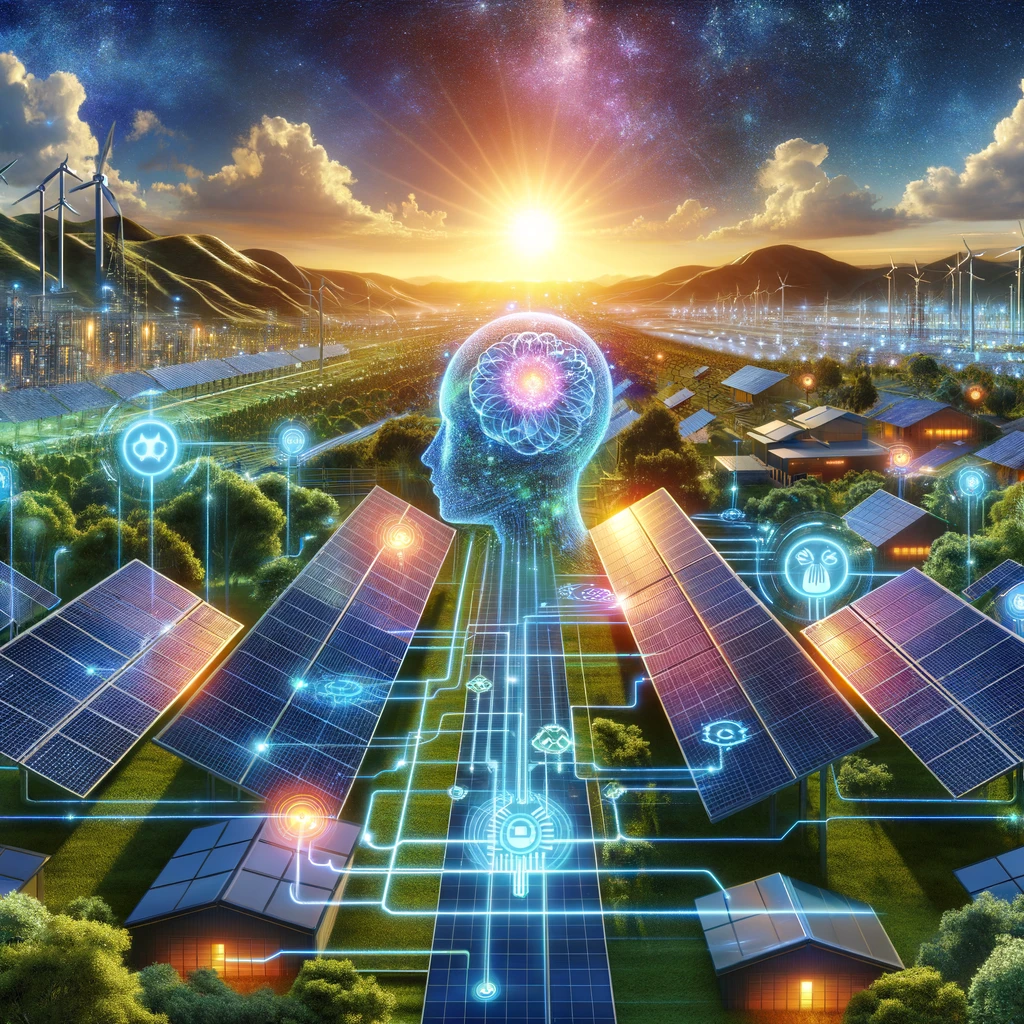This vibrant and futuristic image depicts a striking scene centered around a digital head turned to the left, with a pulsating bright blue brain connected to an advanced network of circuitry. The central figure seems to symbolize enlightenment and connectivity through renewable energy, as blue circuitry lines fan out to numerous houses capped with solar panels. The solar panels, notably lifted above the roofs, are linked by these blue lines, enhancing the theme of energy exchange and modernization.

Set against a dark blue and black sky, the bright sun at the center casts an energizing light, while purples, blues, and white hues add depth and dynamism to the scene. Rolling mountain roofs and lush greenery with trees, shrubs, and well-lit houses filled the bottom third of the composition, creating a harmonious blend of nature and technology.

Flanking the scene are wind turbines, emitting a blue glow and interwoven with the same circuitry, emphasizing the theme of sustainable energy. The entire composition, with its intricate details and vivid colors, woven together with digital elements and natural landscapes, portrays a message of interconnected renewable energy sources leading towards a brighter, enlightened future.